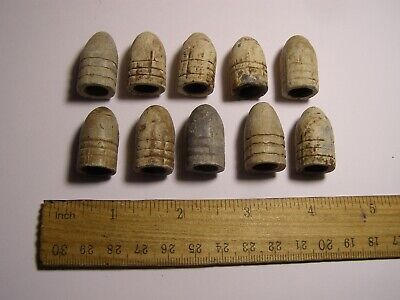The image showcases ten small cylindrical objects, resembling old, weathered bullet tips, organized into two rows of five each. These bullets, marked by grooves around their bases, vary in color from white to copperish or goldish hues, with one dark gray item taking center position in the second row. They are visibly worn and dirty, as if unearthed recently, displaying patches of rust and dirt. Beneath these objects lies an old, dirty, tan-colored wooden ruler, measuring the total width of the bullets in a row to be about four and a half inches. The arrangement rests on an off-white surface with a gradient gray background that fades to a deeper shade, adding a translucent ambiance to the photograph.